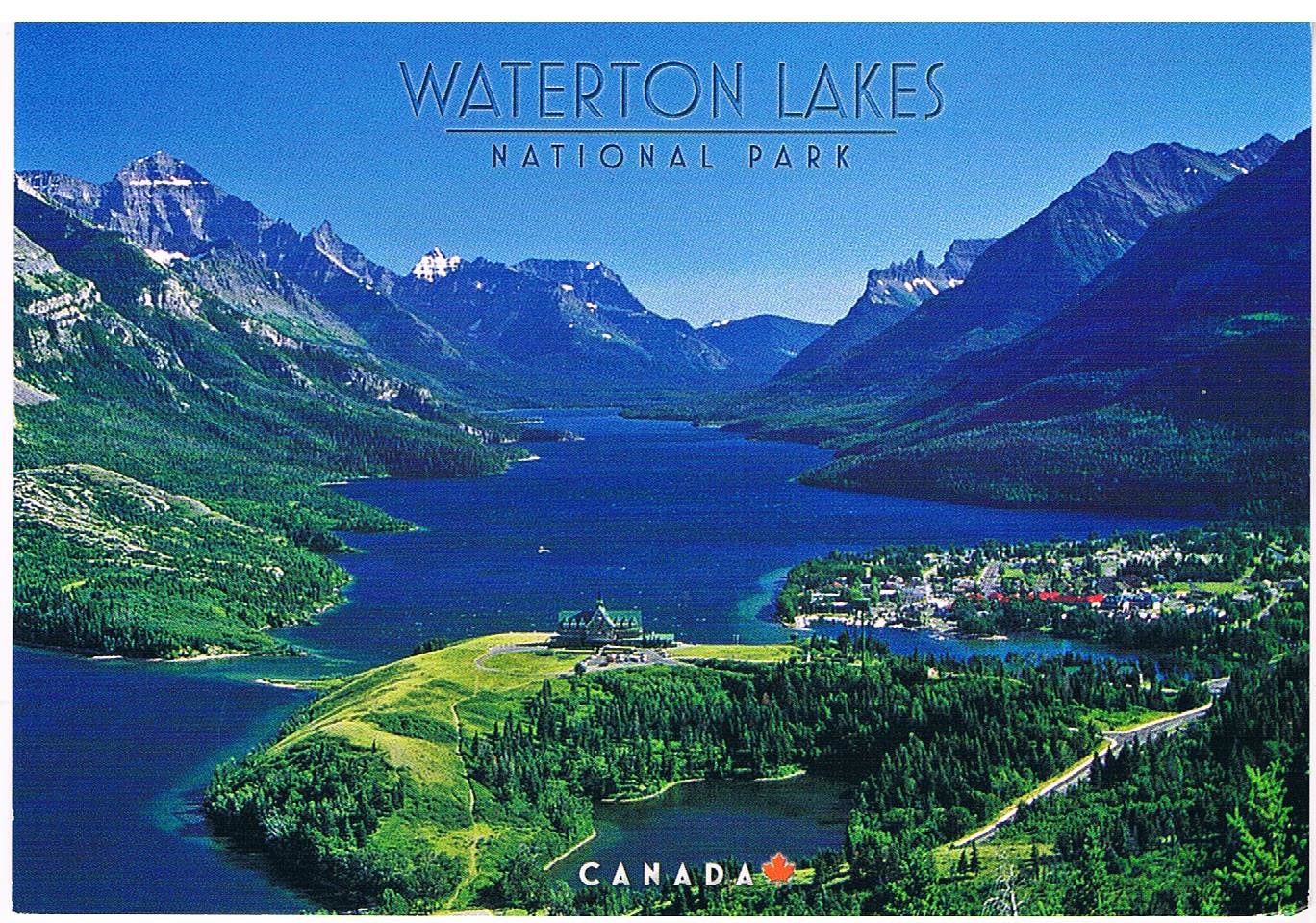This image is an aerial postcard of Waterton Lakes National Park in Canada, showcasing a breathtaking landscape. The vibrant color palette includes shades of blue, light blue, gray, white, green, light green, and red, which vividly highlight various natural and man-made features. At the forefront, a deep blue lake extends from the bottom left and meanders through the center of the image, flanked by lush green land masses on both sides. Surrounding the lake are rolling hills, studded with trees, a light green hill with a prominent mansion in the middle, and various buildings. Further into the distance, majestic mountains with occasional snow-capped peaks frame the scene. At the top of the postcard, the text "Waterton Lakes National Park, Canada" is prominently displayed. The entire postcard, in an outdoor midday setting, fills the photo, emphasizing the expansive and serene beauty of the national park. A road meanders along the terrain, and additional land juts out around the lake, enhancing the composition's depth and complexity.